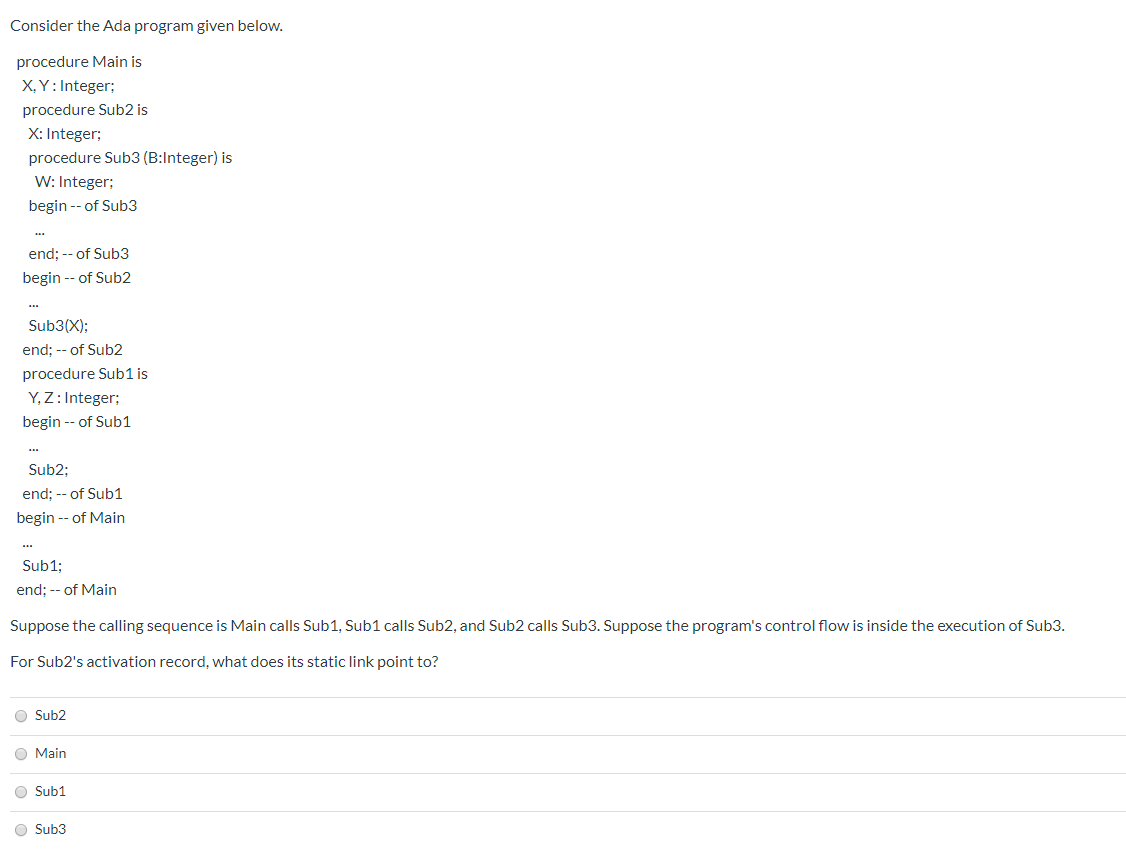A detailed photo caption for the given image might look like this:

---

A screenshot of a programming exercise in the ADA language is displayed. In the top left corner, the heading reads, "Consider the ADA program given below." Beneath this heading, lines of ADA code are arranged vertically down the screen, illustrating a section of a program. At the bottom of the screen, an instruction states: "Suppose the calling sequence is main calls sub 1, sub 1 calls sub 2, and sub 2 calls sub 3. Suppose the program's control flow is inside the execution of sub 3. For sub 2's activation record, what does its static link point to?" Below this question, four possible answers are provided, each accompanied by a selection button. The choices are labeled as: "sub 2," "main," "sub 1," and "sub 3." This setup suggests that the image is part of an online assessment or instructional material for a college-level computer science course.

---